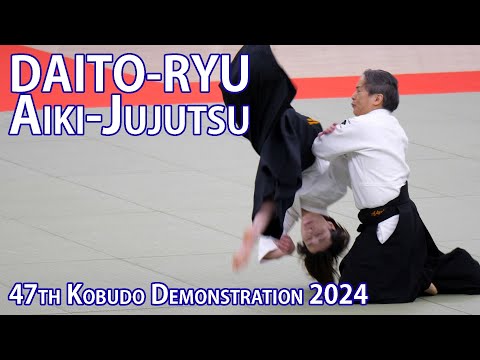The image is a detailed poster for the "47th Kobudo Demonstration 2024," featuring the martial art Daito Ryu Aiki Jujutsu. At the top, "Daito Ryu" and "Aiki Jujutsu" are prominently displayed in white capital letters with a blue outline. The background consists of a grayish-white square flooring design intersected by a red line. The image has black borders on the top and bottom.

At the bottom left, the text "47th Kobudo Demonstration 2024" is also in white with a blue outline. The scene depicts two men in martial arts attire on a gray mat indoors. One man with short, graying dark hair and wearing a white long-sleeve shirt and black pants is kneeling, seemingly mid-action as he flips another man. The other man, who has longer dark hair and is also dressed in a white top and black bottoms, is in mid-air, upside down from the flip.